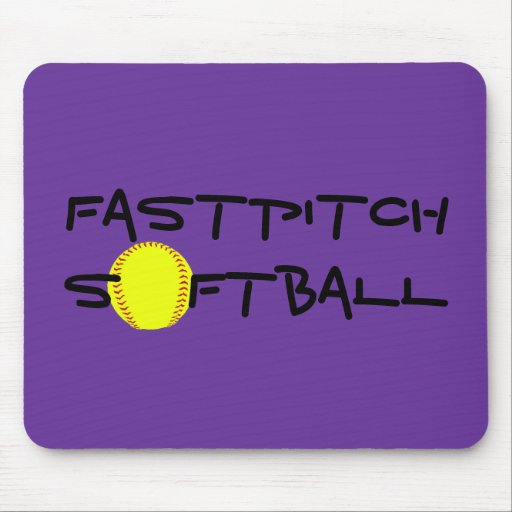In the center of the image, a solid medium-purple rectangular object with rounded edges dominates about 90% of the space, set against a white, wood grain-textured background. This object, resembling a mouse pad, features the phrase "FAST PITCH SOFTBALL" written in a unique, modern, sketch-like font in black capital letters. Notably, the 'O' in "SOFTBALL" is represented by a slightly larger yellow softball with red horseshoe-pattern stitching, adding a vibrant contrast to the design. The layout of the text spans horizontally across the purple surface, with "FAST PITCH" appearing as a combined term above "SOFTBALL," suggesting a close connection to the sport, possibly for someone associated with a fast pitch softball league or school team.